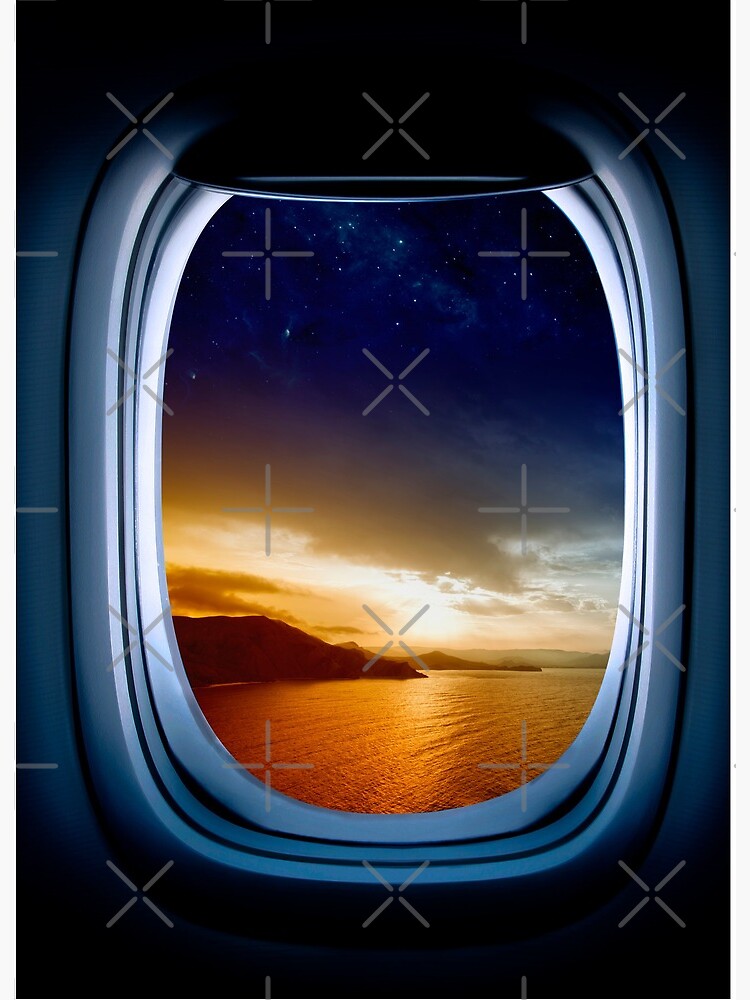The image captures a breathtaking scene through a porthole, which could belong to either an airplane or a cruise ship, given its features. The porthole is a rectangular window with rounded corners and a rubber-like, silver and blue seal. The view outside reveals a stunning sunset over a golden-tan body of water, with majestic mountains in the background. The sky transitions from deep blue at the top to shades of orange, pink, and white near the horizon, where the sun has just set. There are dark clouds and the beginning of nightfall, with a few stars peeking through. Multiple light gray X’s and pluses watermark the image, likely to prevent unauthorized copying. The whole scene is set against a blue background, enhancing the serene, picturesque quality.